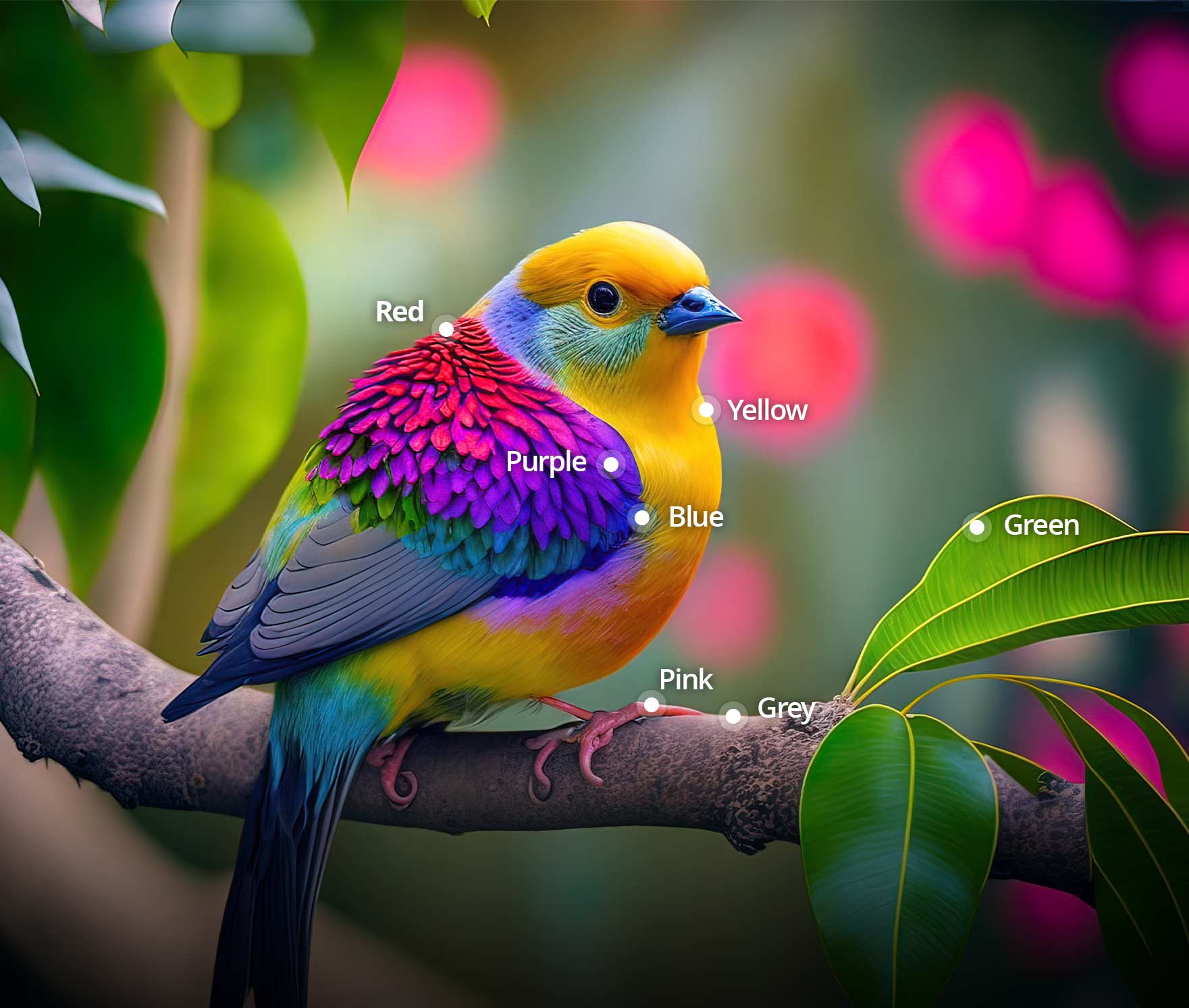This is a dramatically colored and vibrantly detailed photograph of an extraordinarily colorful bird perched on a slightly curved, brown, and purplish branch that spans from left to right. The background is blurred, featuring a pastel green surface with bright pink spherical elements that resemble flowers. The branch is adorned with striking, vibrant green leaves with yellow veins located towards the right of the image.

Perched elegantly on the branch, the bird's plumage showcases a vivid array of colors. Its talons are pink, and the bird's tail is black with shades of blue, lime green, and yellow on top. The breast displays a bold orange and yellow hue, transitioning to red, purple, and blue on the wings, which end in gray and dark blue wingtips. The bird's head is topped with bright yellow feathers, complemented by a blue and light blue neck. The deep, shiny black eye and sharp blue beak add to the bird's striking appearance.

Additionally, the image features textual labels in white dots, marking the various colors on the bird and its surroundings. These labels include "red" at the top of the wing, "purple" on the right side of the wing, "blue" beneath that, "yellow" on the chest, "pink" on the talons, "gray" on the branch, and "green" on the leaves. The meticulous labeling and the bird's vibrant, almost surreal coloration suggest a possible photoshop enhancement, adding to the image's overall dramatic and intricate presentation.